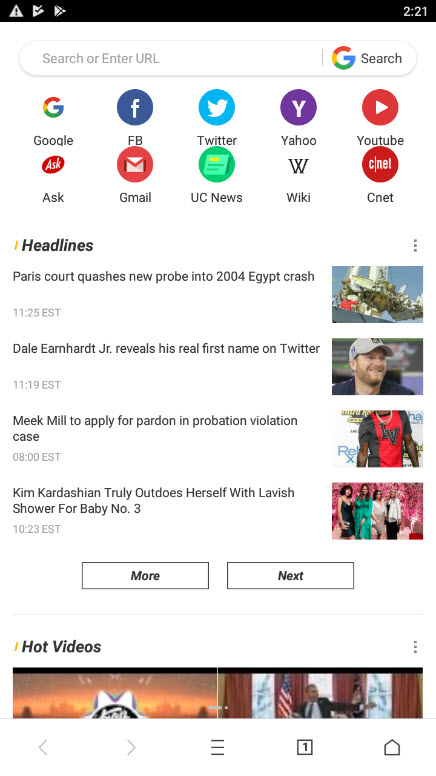This image depicts the Google homepage as viewed in the Google app on an Android cell phone. The page shown is the default home screen that appears upon opening the Google search app or browser. 

At the top of this homepage are shortcuts to frequently used or suggested websites for quick access. These shortcuts include popular sites such as Google, Facebook, Twitter, Yahoo, YouTube, Ask.com, Gmail, UC News, Wikipedia, and CNET.

Beneath these shortcuts, the screen displays a series of headlines from various news stories, reflecting a blend of different news categories. The top headline reads, "Paris Court Quashes New Probe Into 2004 Egypt Crash." The second headline announces, "Dale Earnhardt Jr. Reveals His Real First Name on Twitter." Following that, the third headline states, "Meek Mill to Apply for Pardon in Probation Violation Case." The fourth headline shares a piece of celebrity news: "Kim Kardashian Truly Outdoes Herself with Lavish Shower for Baby Number Three."

The headlines illustrate a mix of world news, national updates, and entertainment gossip, catering to diverse reader interests.